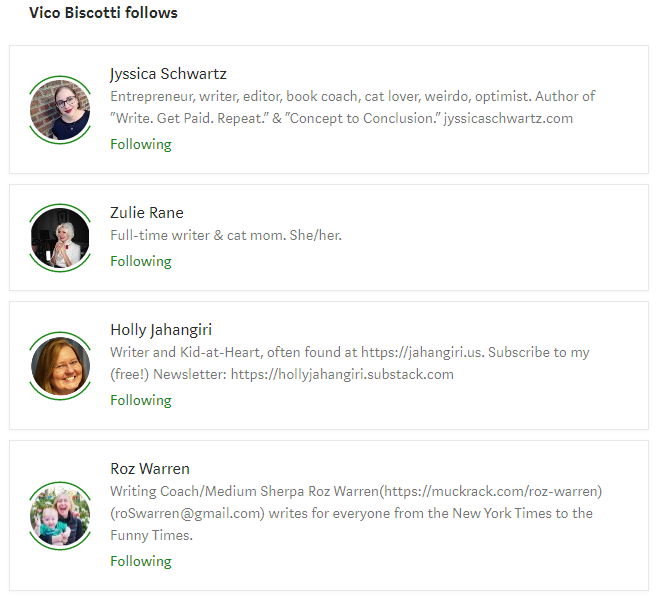Screenshot of a social media app interface against a white background, featuring a list of accounts followed by Vico Biscotti. Each account is enclosed in a light gray thin rectangular border and includes detailed descriptions alongside profile pictures:

1. **Jessica Schwartz** (spelled J-Y-S-S-I-C-A Schwartz): 
   - Profile Picture: Woman wearing a black shirt, bright red lipstick, posing against a brick wall.
   - Description: Entrepreneur, writer, editor, book coach, cat lover, weirdo, optimist, author of "Write, Get Paid, Repeat" and "Concept to Conclusion". 
   - Website: JessicaSchwartz.com
   - Status: Following (indicated by a green button).

2. **Zulie Rayne** (spelled Z-U-L-I-E-R-A-N-E):
   - Profile Picture: Person with white hair wearing a white shirt, with a black background.
   - Description: Full-time writer and cat mom. Pronouns: she/her.
   - Status: Following.

3. **Holly Jangiri**:
   - Profile Picture: Close-up of a woman's smiling face with light brown hair.
   - Description: Writer and kid at heart, often found at jangiri.us. 
   - Newsletter: Subscribe to my free newsletter at https://hollyjangirisubstax.com.
   - Status: Following.

4. **Ros Warren**:
   - Profile Picture: Person holding a baby with greenery in the background.
   - Description: Writing coach, Medium Sherpa. Writes for everyone from The New York Times to The Funny Times.
   - Email: RosWarren@gmail.com (in brackets).
   - Website: muckrack.com/RosWarren
   - Status: Following.